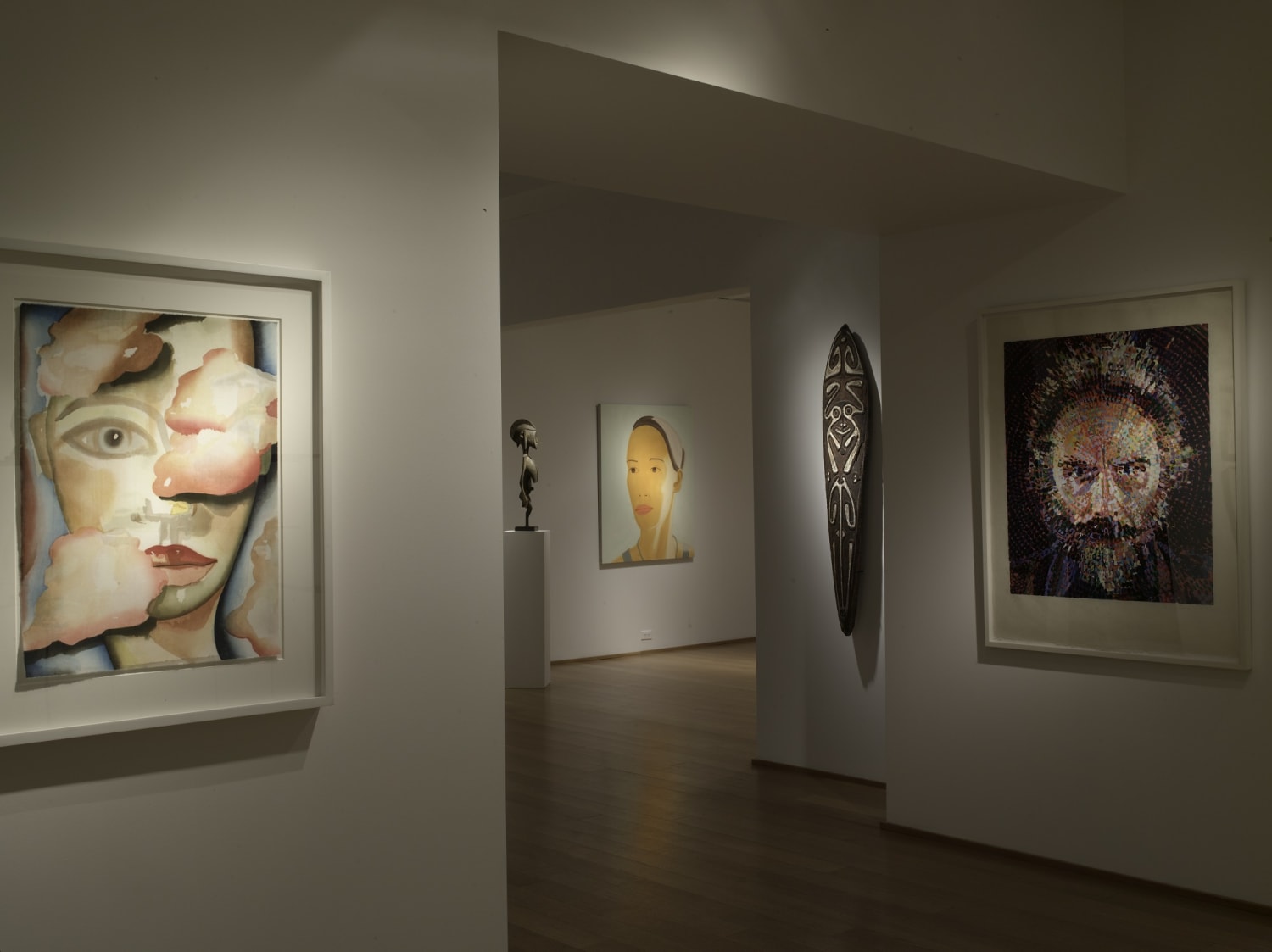The photograph captures the interior of an art gallery exhibiting multiple pieces of modern artwork. Predominantly white walls create a minimalist backdrop within the dimly lit space, with strategic lighting highlighting specific works. To the left, an abstract drawing portrays a partial human face featuring the right eye, red lips, and the left eye and forehead. This piece is surrounded by three pink patches that add an unusual and surreal element to the composition. 

In contrast, the wall on the right showcases a similarly abstract yet distinctly different image of a man. Rendered in a pointillist style with intricate dots, this depiction shows a serious-looking man with a black mustache against a dark background, giving the piece a somber and intense atmosphere. Adjacent to these artworks, a hallway extends into another room, displaying a sculpture and additional art pieces, which provide depth and further intrigue in the overall gallery setting.